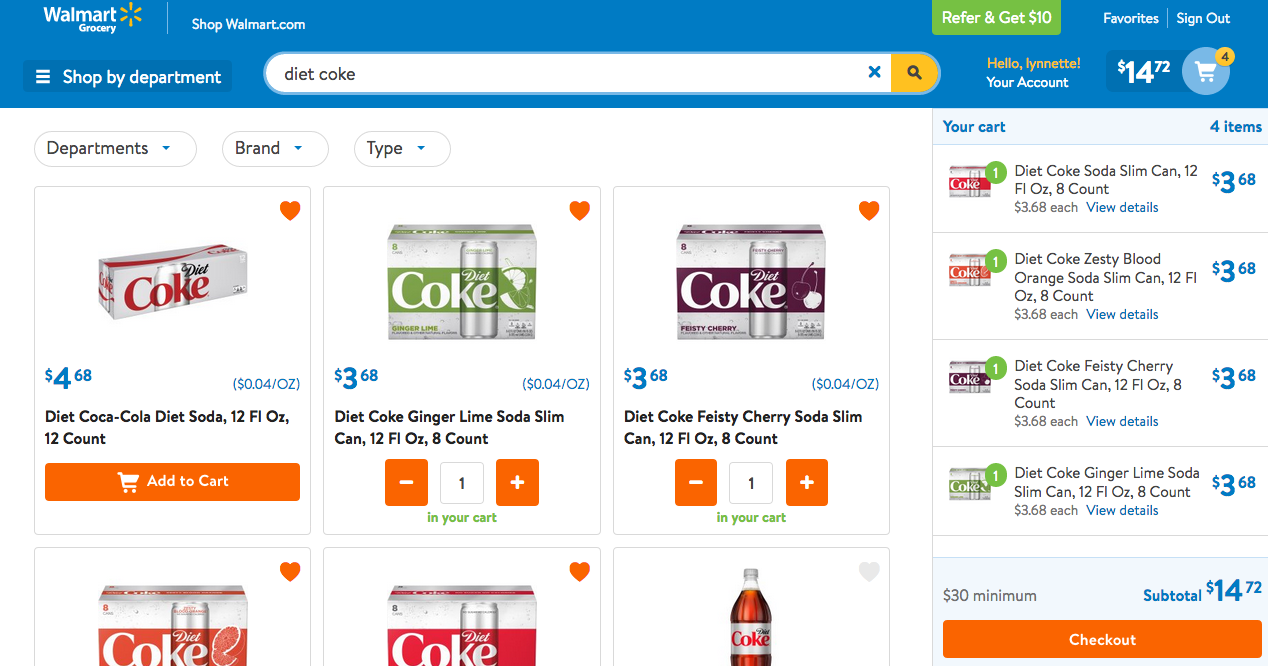This image showcases a Walmart Grocery webpage, featuring a user interface designed for shopping. At the top, a blue banner stretches across the screen, prominently displaying "Walmart Grocery" on the upper left. Adjacent to this, the website URL "Shop Walmart dot com" is located. On the right side of the banner, a green rectangle with white text offers a referral bonus: "Refer and get $10." Nearby, options for "Favorites" and "Sign Out" are visible.

Beneath the banner, the page presents a "Shop by Department" section. Centered within this section is a white oval search bar, into which the user has typed "Diet Coke." A greeting, "Hello Lynette, Your Account," is placed nearby, along with an icon indicating a shopping cart containing four items totaling $14.72.

The main content area displays search results for various types of Diet Coke, listing six different product options. The right side of the page features a mini cart summary, detailing the selected items. The items in the cart include:
1. Diet Coke Slim Can
2. Diet Coke Zesty Blood Orange Soda Slim Can
3. Diet Coke Feisty Cherry Soda Slim Can
4. Diet Coke Ginger Lime Soda Slim Can

An orange rectangle at the bottom invites the user to proceed to checkout.